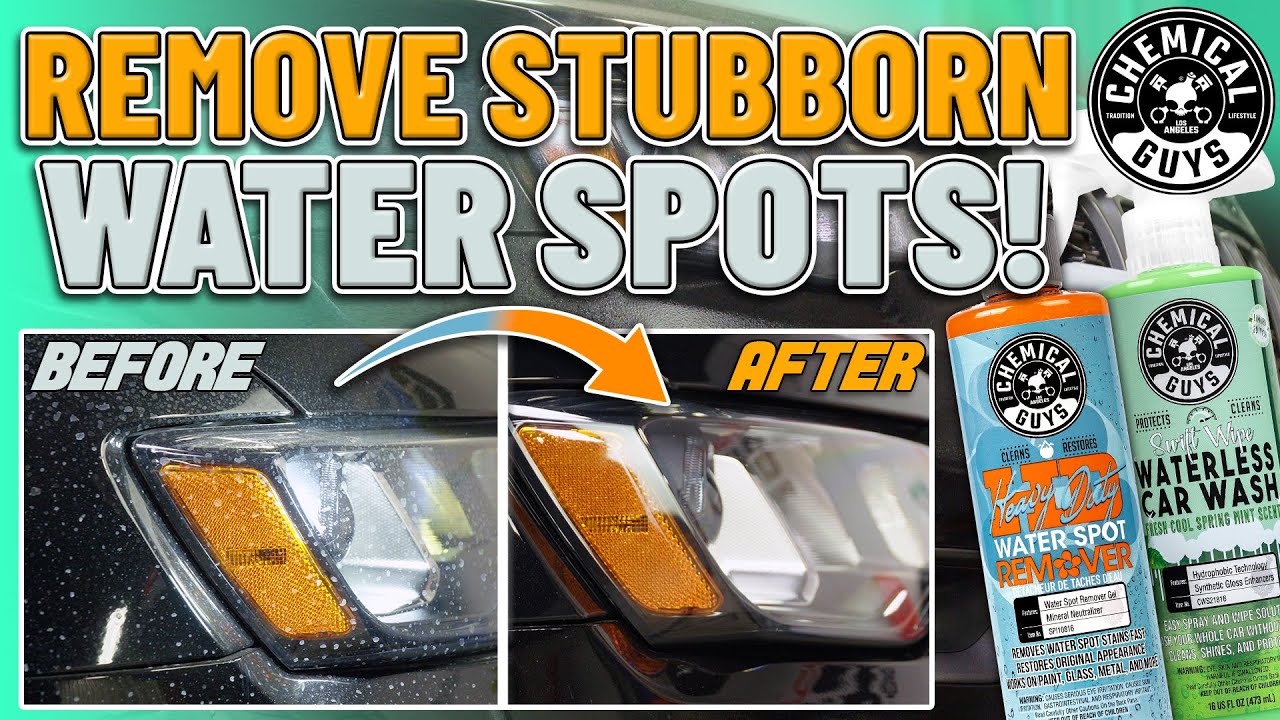The image is a detailed advertisement for car cleaning products by Chemical Guys, prominently featuring two plastic bottles in the bottom right corner and two overlaid circular logos that say "Chemical Guys." The products highlighted include a green bottle labeled "Swift Wipe Waterless Car Wash Cool Spring Mint Scent" and a blue bottle with an orange label that says "Heavy-Duty Water Spot Remover." At the top left, bold text reads "Remove Stubborn Water Spots!" with an exclamation point. Below this headline, a before-and-after comparison is illustrated: on the left, a photo of a black car's front fender and headlight lens shows visible water spots and lime spots caused by sun-drying, marked with the word "before." An arrow points to the right towards another image labeled "after," showing the same black car, now spotless and clean. This comprehensive advertisement demonstrates the effectiveness of the products in removing persistent water spots and enhancing car appearance.